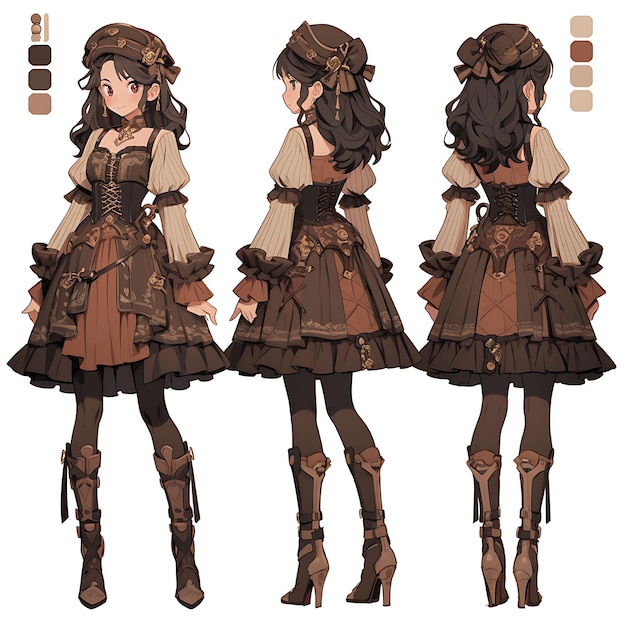The image is a detailed digital illustration of an anime-style girl set against a white background. The artwork features her in three different positions: from the front, back, and a slanted back view. She has long, flowing brown hair and large, expressive red eyes, with a brown headgear that includes a bow visible from the rear view. Her outfit is a medieval-themed, multi-shaded brown corset dress paired with a white puffy-sleeved shirt, detailed with brown and orange accents at the cuffs. The dress has a layered, short skirt combined with brown tights. She is also sporting knee-high, high-heeled boots, which have scabbards for knives. Additionally, she wears a necklace, adding to her medieval flair. The corners of the image display color palettes with various shades of brown, allowing for customization. The overall attire is accentuated with belts and corset lacing, emphasizing the intricate design.